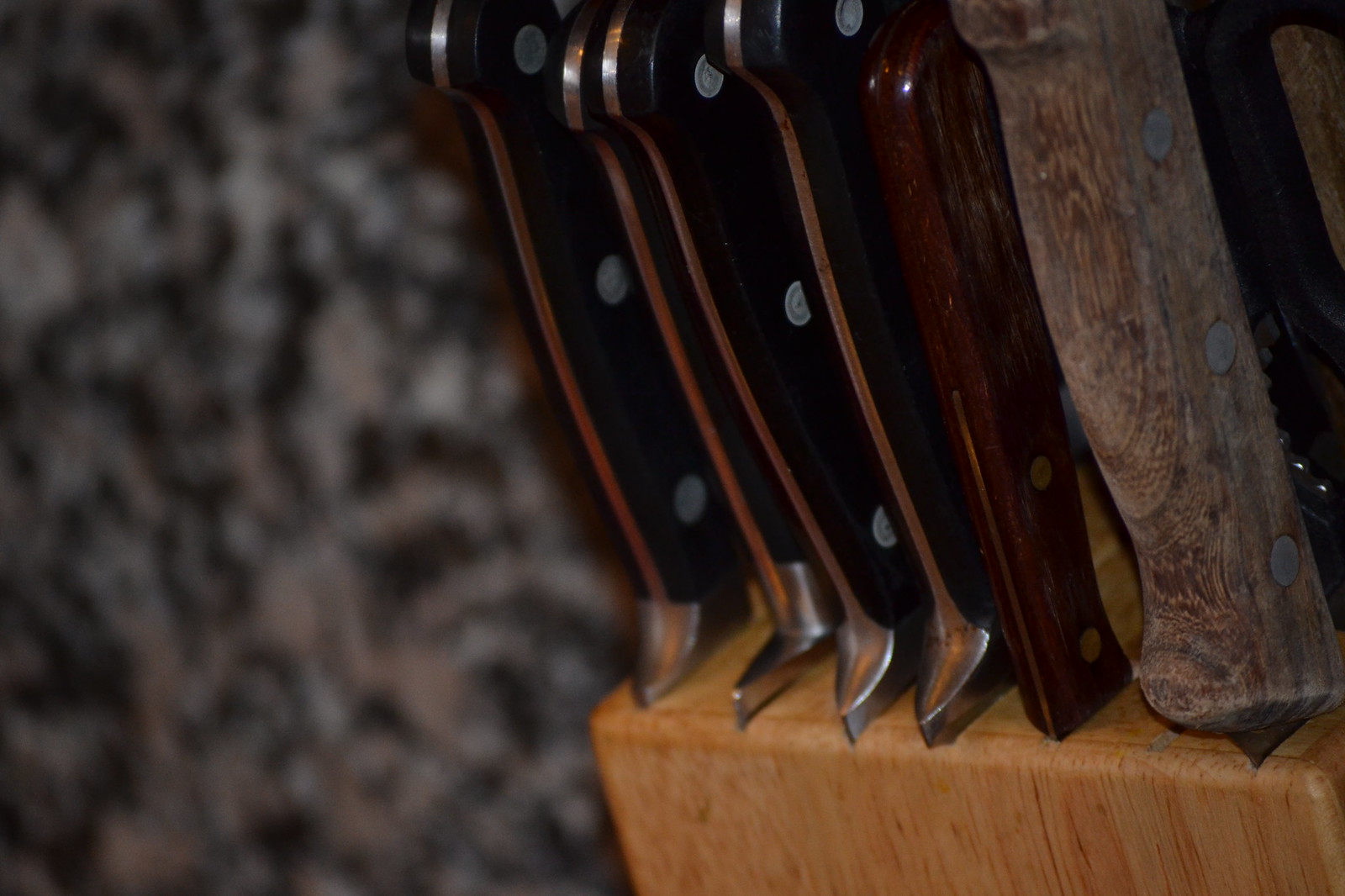This close-up photograph showcases a wooden knife block prominently positioned in the bottom right corner of the image. The background on the left is a blurred gray, preventing any discernible details. The knife block itself is a square of light-colored wood with multiple slots on top, where six knives are inserted. The first four knives, oriented from left to right, feature silver stainless steel blades and black plastic handles adorned with three silver circles each. Following these, a fifth knife stands out with a dark brown wooden handle, suggesting it's stained or treated. The sixth knife sports a thicker handle made from light-colored, untreated wood, giving it a handmade appearance. The overall composition and varied handle materials provide an intriguing contrast against the muted background.